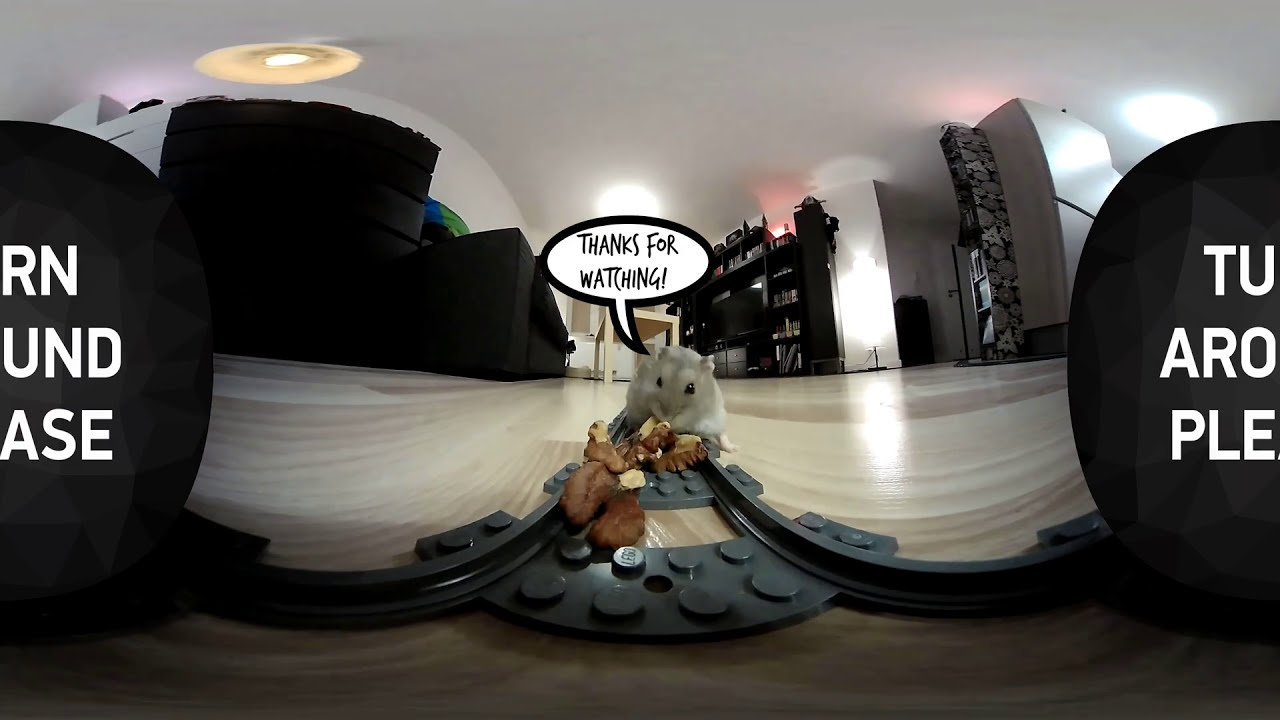The panoramic 360-degree image showcases a whimsical scene that appears to combine photography with graphic elements. Dominating the foreground is a large round black graphic object bisected such that one side bleeds off the right edge and the other off the left. The graphic has the phrase "TURN AROUND PLEASE" in bold white uppercase text, split between the two halves. At the center of the image, a small rodent, possibly a mouse or hamster, stands on what resembles a Lego train track, complete with plastic rails and flat Lego brick ties. Scattered around the track are what appear to be nuts or dried fruit, which the mouse is interacting with. Above the mouse is a thought bubble with the text "Thanks for watching." The background features a linoleum or hardwood floor, possibly part of a home or apartment. Further back, an entertainment center with a TV and various media sits against a white wall, and a black couch can be seen to the left. The overall effect combines elements of VR 360 imaging with playful and surreal touches, merging real and graphic elements seamlessly.